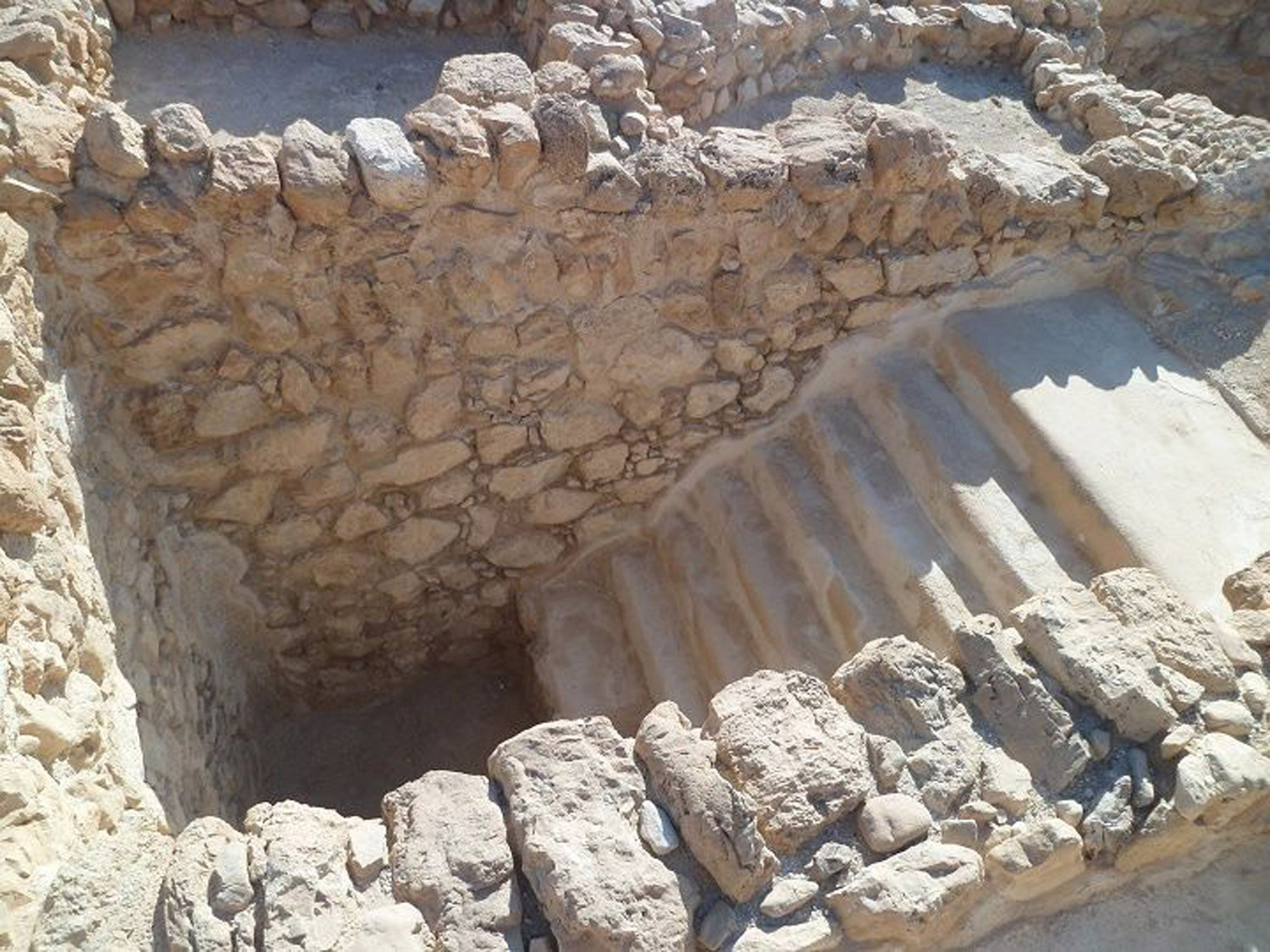This horizontal rectangular image captures a photograph of what appears to be ancient ruins, specifically showcasing a well-worn concrete staircase descending into a small, almost prison-like pit. The stairs are very smooth and polished, in contrast to the rough, light tan-colored stone walls that surround them. These walls are held together with some sort of brownish mortar. At the top of the stairs, part of another room extends along the uppermost wall, giving a glimpse of further architectural complexity. On the left side at the top, there's another adjoining room with thick stone walls, suggesting significant structural integrity. The overall scene hints at the remains of what could have been a mine, temple, or similarly ancient and significant site, characterized by its rock and stone construction and the intricate interweaving of steps and spaces.